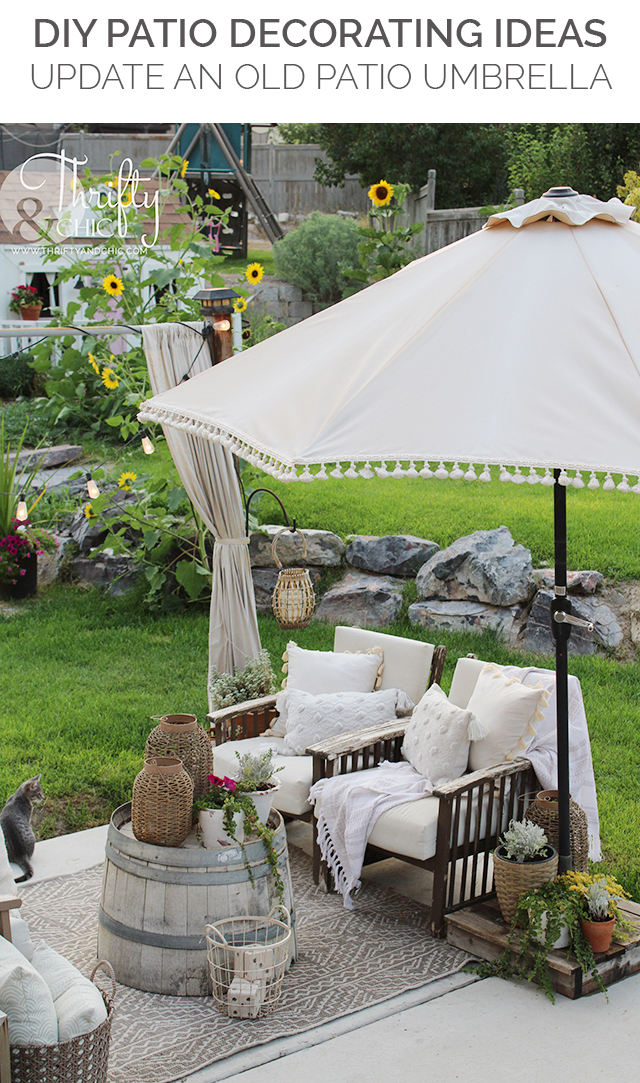This image, seemingly a cover of an advertisement or flyer, prominently features the text "DIY Patio Decorating Ideas: Update an old patio umbrella" in black at the top. The scene showcases a well-maintained garden with green grass and a variety of plants, including sunflowers in the background. A border made of large stacked rocks separates the lawn from a patio area. Central to the scene is an old patio umbrella, updated with a fringe around its edge, providing shade over two wooden chairs with white cushions, which are accompanied by a rug on a cement surface. An artsy and crafted vibe is depicted with several potted plants, woven containers, and baskets. An overturned barrel serves as a quirky table. A small gray cat is seen exploring the area, adding a charming touch to the garden's serene atmosphere. The text "Thrifty Chick" is noted in the top left corner of the image.